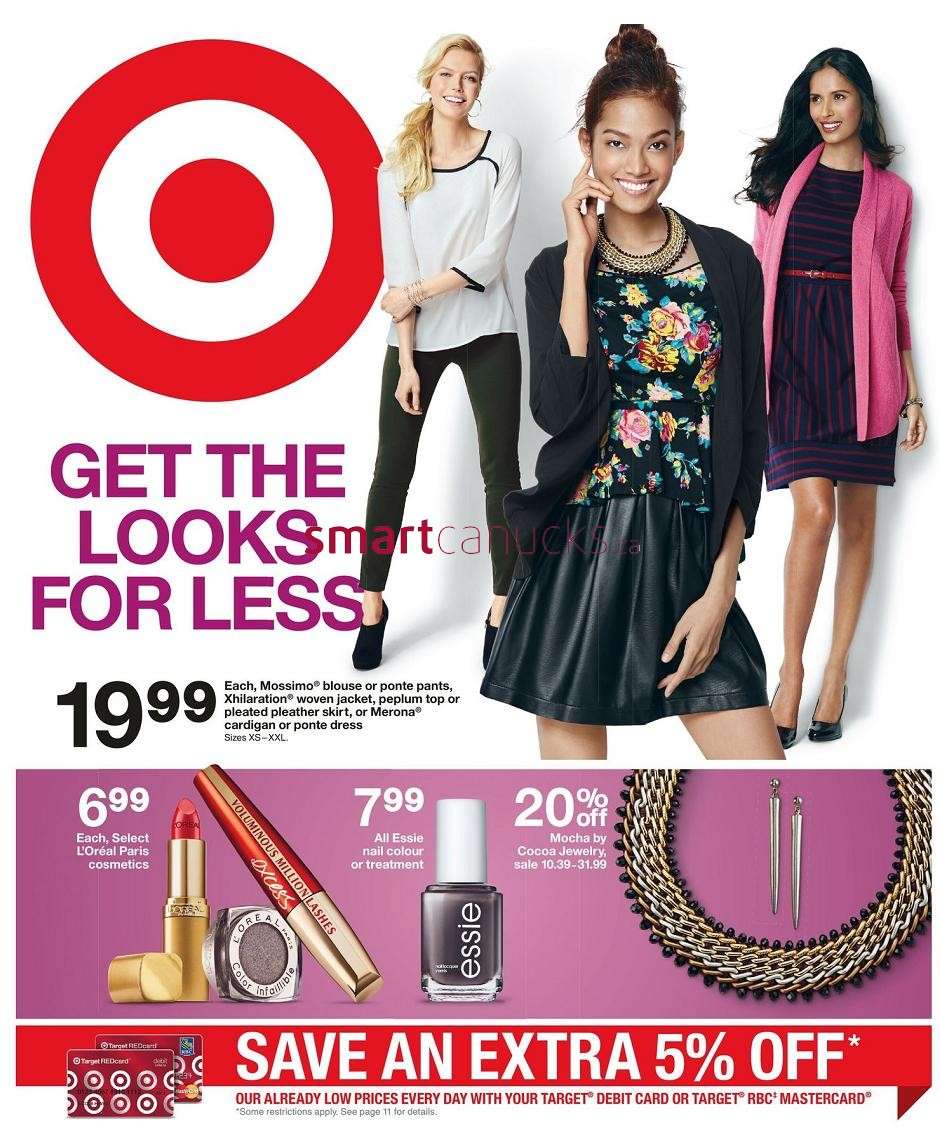**Front Page of a Target Sales Ad**

The front page of this Target sales ad features a clean, white background with the iconic red Target logo prominently displayed in the top left corner. Below the logo, in a pink font, are the words "Get the looks for less."

The top right section of the ad showcases three women modeling fashionable outfits. The first woman has blonde hair and is dressed in a white shirt trimmed in black, black pants, and black high heels. The second model sports a black skirt, a black and floral print shirt under a black cardigan, and has reddish-brown hair. The third woman is seen wearing a blue and pink striped dress paired with a pink jacket and black high heel shoes, complemented by her long black hair.

Prices for the featured clothing items are prominently displayed, stating "$19.99 each." The text lists various items such as Massimo Blouse or Panty Pants, Exhilaration Woven Jacket, Peplum Top or Pleated Leather Skirt, and Morona Cardigan or Panty Dress.

Below the outfits, three additional products are displayed: L'Oreal lipstick, nail polish, and a stylish necklace. At the very bottom of the ad, consumers are reminded of the savings they can achieve with the text: "Save an extra 5% off our already low prices every day with our Target Debit Card or Target RBC Mastercard."